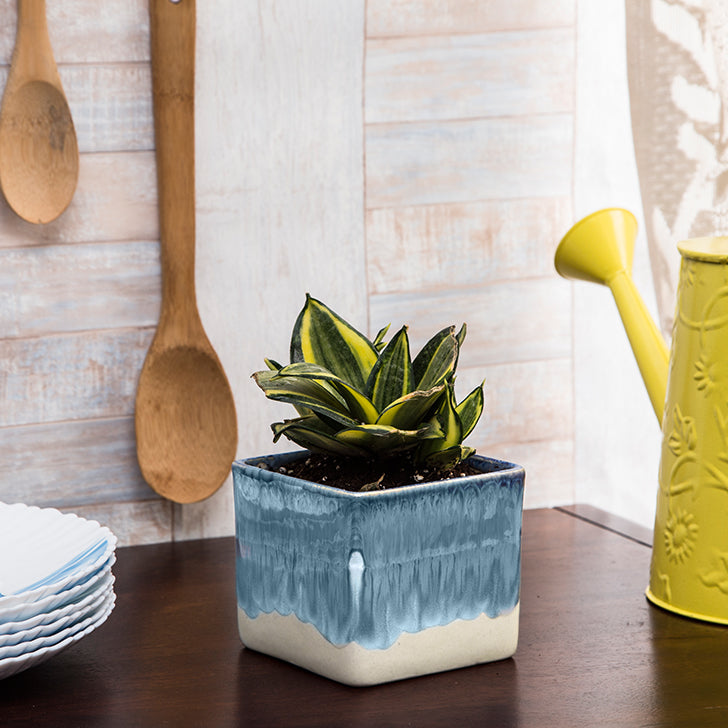This image showcases a cozy sunroom scene centered around a dark brown wooden table. On the table lies a small, square planter, featuring a blue top and a white base, containing a single green succulent nestled in planting soil. To the left of the planter, there is a stack of six blue and white scalloped plates, resembling seashells. To the right, near the edge of the table, stands a clean, glossy yellow tin watering pail adorned with raised floral patterns. The background consists of a textured wall with a cottage-colored pattern, and hanging in the top right against the wall are two wooden spoons. The scene is bathed in red light coming from the top right corner of the image, adding a warm touch to the setting.